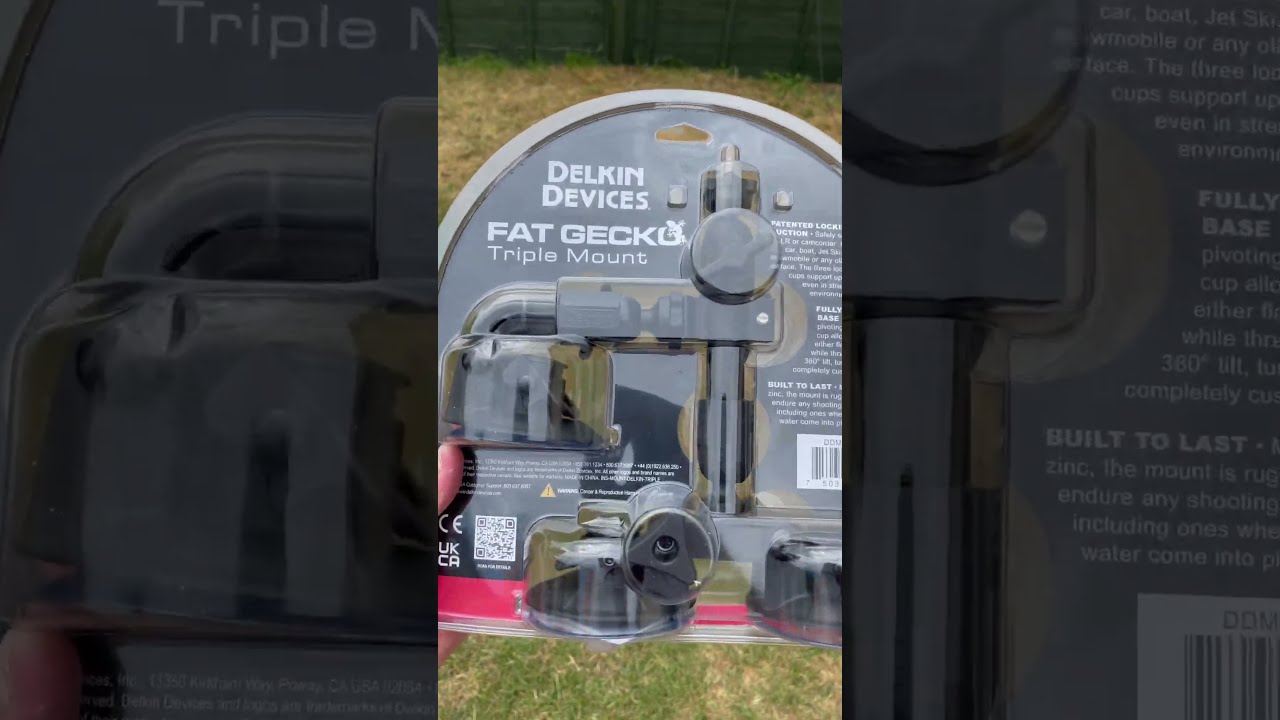The photo features a person holding a Delkin Devices Fat Gecko Triple Mount in its clear, hard plastic packaging. The device, intended for mounting, is encased in a form-fitting transparent cover that reveals its gray components and distinctive triple mount design. The packaging prominently displays "Delkin Devices" in the upper left corner, followed by "Fat Gecko Triple Mount" underneath. The hand holding the package is visible on the left side of the image, with a grassy lawn serving as the backdrop, indicating the photo was taken outdoors. Additional details on the package include a QR code on the left and a barcode on the right. The background is dark gray with shadowed edges, emphasizing the product in the center, which also features text on the right that reads, “Built to Last.”